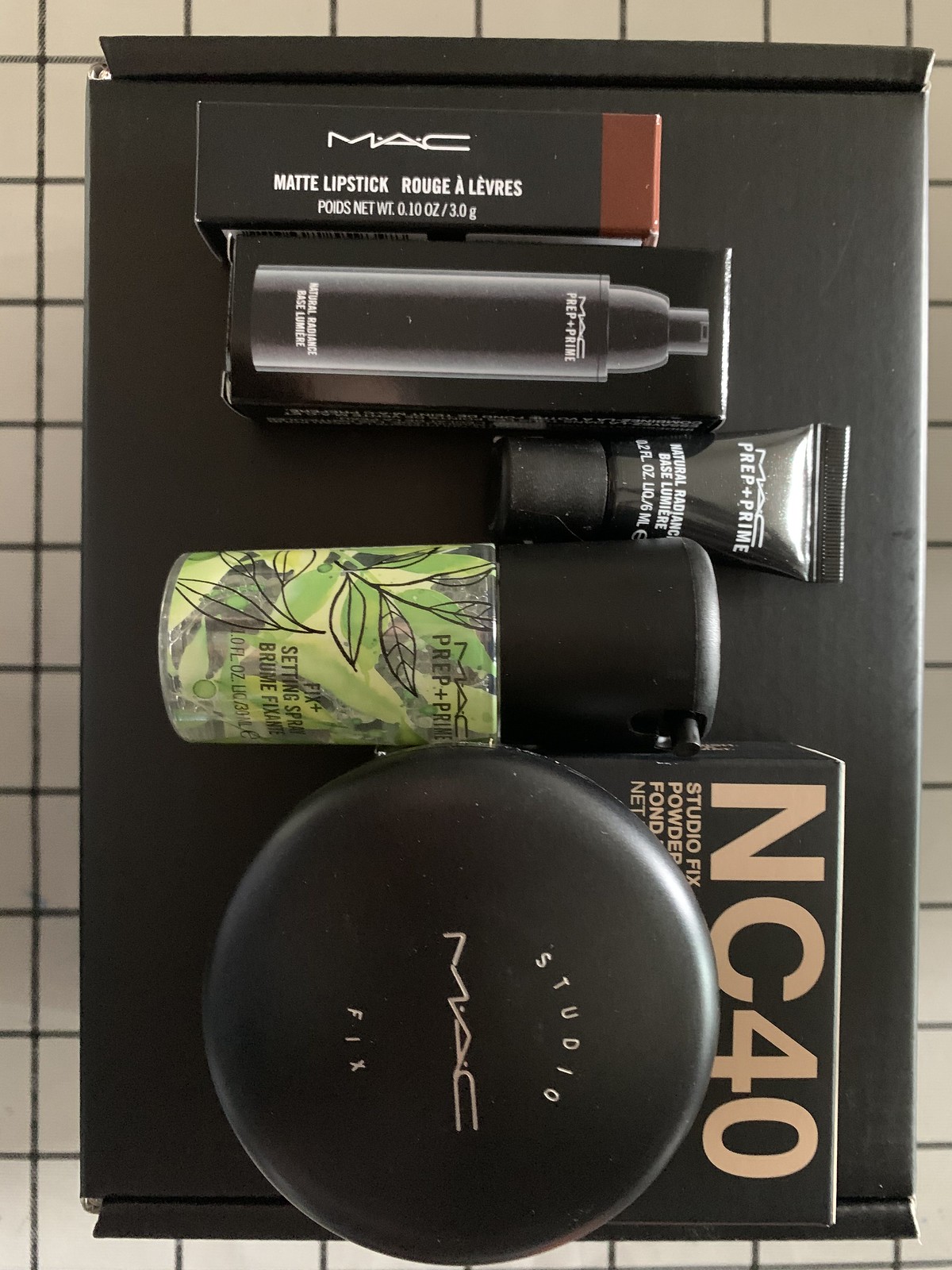The image showcases an assortment of beauty products from the renowned makeup brand MAC. All the items are neatly arranged on a black cardboard box, likely the original shipping container. 

At the top of the arrangement, there is a sleek, black rectangular cardboard box with a subtle reddish-brown tip. The box is labeled in white text as "MAC Matte Lipstick," indicating a net weight of 0.1 ounces or 3 grams.

Directly below this, a black rectangular package features an image of a bottle and is labeled "MAC Prep + Prime Natural Radiance." This package is followed by a smaller black squeezy plastic container, also part of the "MAC Prep + Prime Natural Radiance" line.

Further down, a glass container with a beautiful design of green leaves outlined in black catches the eye. It has a black cap and an integrated pump top. Though the container is slightly turned, the visible text reads "MAC Prep + Prime Fix+ Setting Spray."

Continuing down the arrangement, there is a large black circular compact labeled "Studio MAC Fix," which might be a typo as it should read "MAC Studio Fix."

At the bottom, a box labeled "NC40 Studio Fix Powder" completes the collection, possibly the packaging for one of the aforementioned products.

This detailed composition of MAC beauty products not only highlights the variety but also the elegant design and packaging of the brand's offerings.